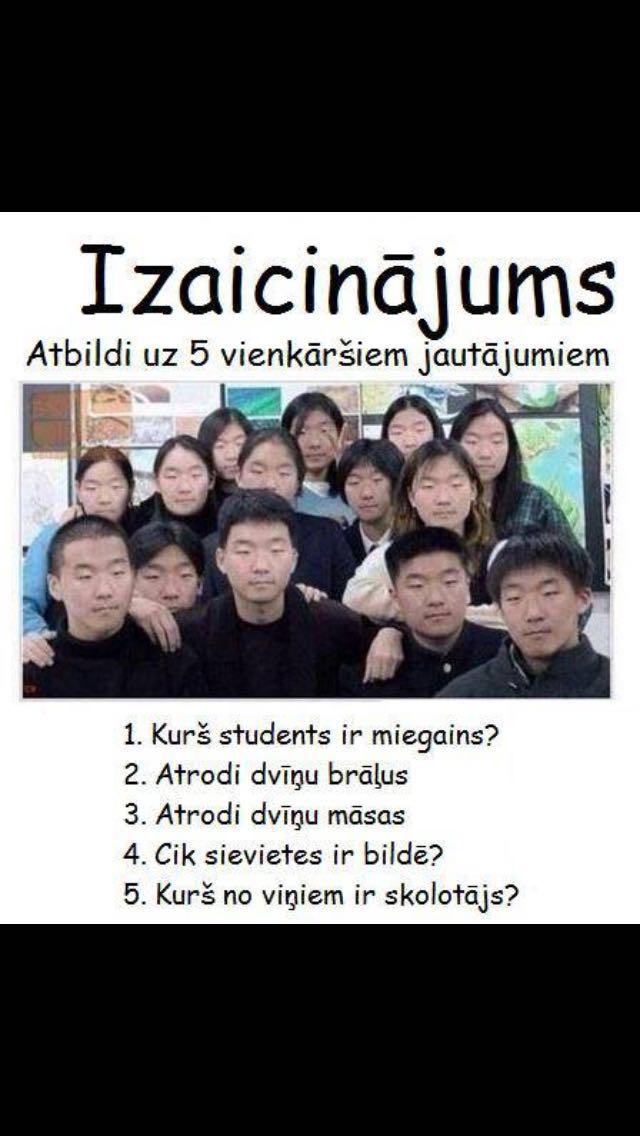The image appears to be a poorly photoshopped and possibly problematic meme, featuring a group of people, both men, and women, all with the same face, notably of Asian descent. The photo is centrally placed within a PowerPoint slide, using the Comic Sans font. Above and below the image are black bars suggesting the image was reformatted to fit a specific size. The group photo shows individuals predominantly wearing black shirts, with one person in a gray jacket over a red shirt and another in a turquoise shirt. There's a significant amount of text in an unintelligible language, with some noticeable words like "IZAICINAJUMS." Underneath the image, there are five numbered questions also in this foreign language. The background of the slide is entirely black, framing the white-centered photo that displays this altered and photoshopped group in front of a segmented window and adjacent to a dark brown wall.